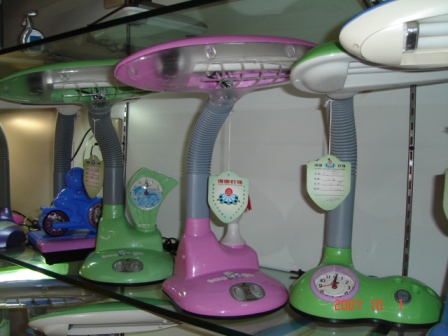The image showcases an assortment of colorful lamps displayed on a glass shelf with a black frame. The lamps, which appear suitable for a child's room, come in pink and light green varieties and all share a similar structure. Each lamp consists of a base, a grayish adjustable stem, and a wide oval-shaped top that encases a light. The base and top are either green or pink, matching the overall theme. The lamps have tags attached, likely indicating prices. In the background, there are beige and white walls. Additionally, a watermark in the corner reads "2007-10-1" in orange lettering, suggesting when the photo was taken. A second glass shelf can be seen above the lamps, adding to the organized display.